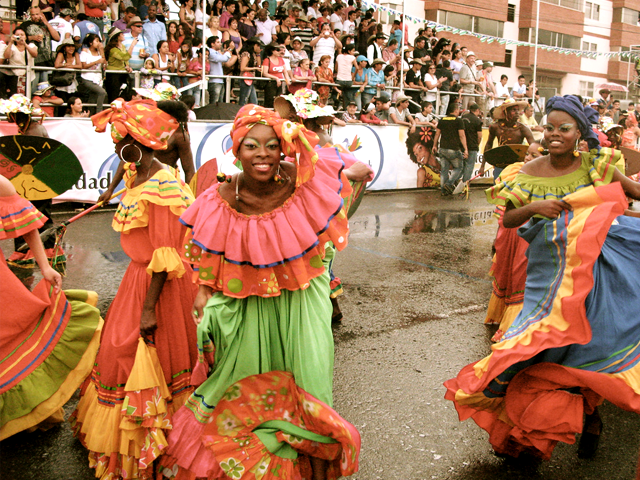The photograph captures a vibrant street celebration featuring a group of joyous, African women in bright, cultural outfits, dancing amidst a wet street with puddles. Their eye-catching costumes radiate a mix of green, red, blue, and yellow, complemented by gorgeous, colorful eye makeup. Accompanying them are a few gentlemen dressed in shorts, hats, and small shields. Both the dancers and the onlookers, who line the sides of the street and stand on balconies of a nearby apartment building, exude happiness and engagement. This energetic parade, advancing from right to left, showcases a beautiful blend of heritage and community spirit as performers move gracefully through the rain-kissed streets, their movements observed and celebrated by the cheerful crowd.